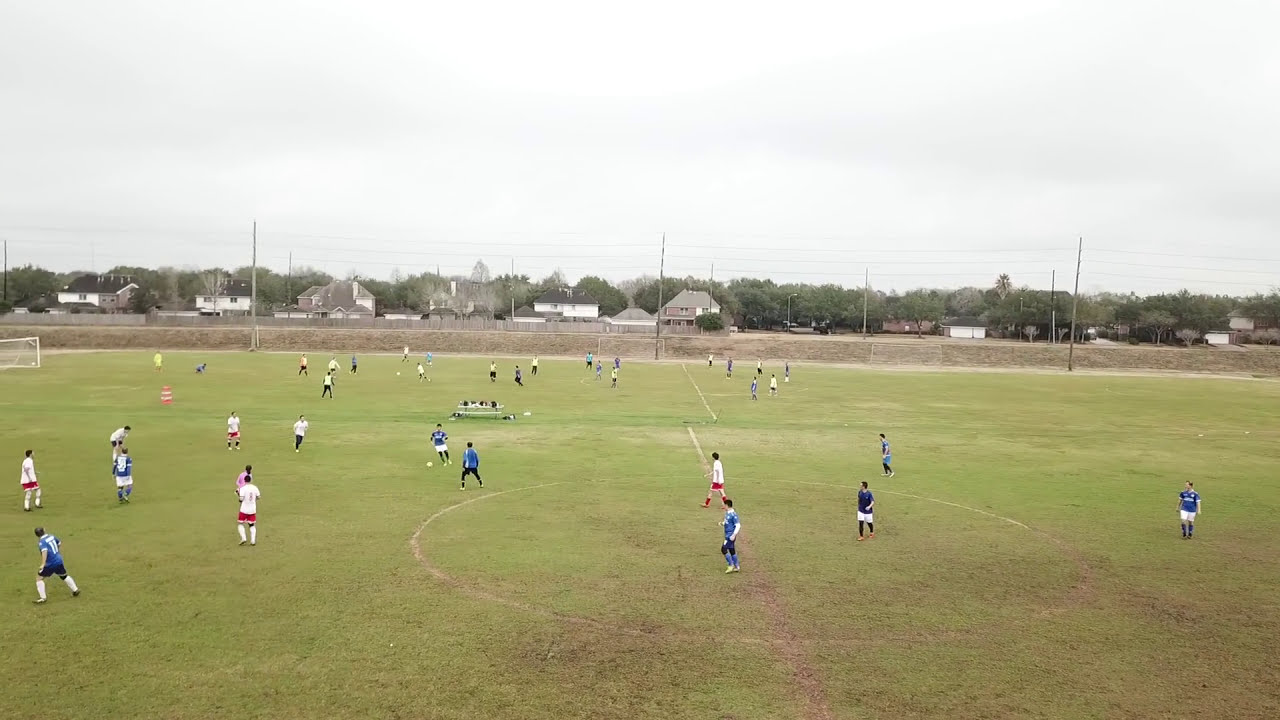The image depicts a lively outdoor scene on a cloudy day, focused on a large grass soccer pitch where approximately 12 players from two opposing teams are actively engaged in a soccer match. One team is outfitted in blue uniforms with black shorts and socks, while the other team wears white shirts paired with red shorts and socks. The midsection of the field shows signs of heavy use, with patches of dirt visible amidst the grass. The match is being officiated by two referees, ensuring the game's fairness. In the background, there is a second adjoining soccer field hosting another match, highlighting that this area comprises multiple sports fields located close to each other. Beyond the fields is a residential area, where a row of houses and buildings is set against a backdrop of green trees and a gray, overcast sky. A wall appears to separate the soccer fields from these residential structures, emphasizing their proximity in this suburban landscape.